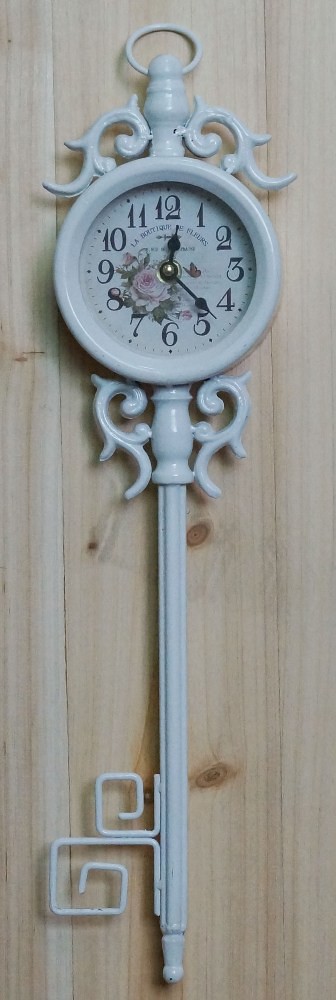This image features a uniquely designed clock shaped like an old-fashioned key, crafted from metal and coated in a light blue color. At the top of the clock, there's a loop for hanging, accompanied by an intricate scalloped metal design. The scalloped pattern continues beneath the clock face, adding a delicate touch to the overall aesthetic.

The clock face itself is white and adorned with a pink flower, creating a beautiful contrast against the blue background. The hours are marked from 12 to 11, with black hands indicating the time.

Supporting the clock is a handle-like structure with a tubular design that is scalloped on the sides, leading down to a long, slender pole that mimics the shaft of an antique key. At the end of the pole, two metal pieces extend, emulating the bit and cleft of an old key, and it concludes with a rounded end. The thoughtfully detailed and whimsical design merges functionality with decorative artistry.